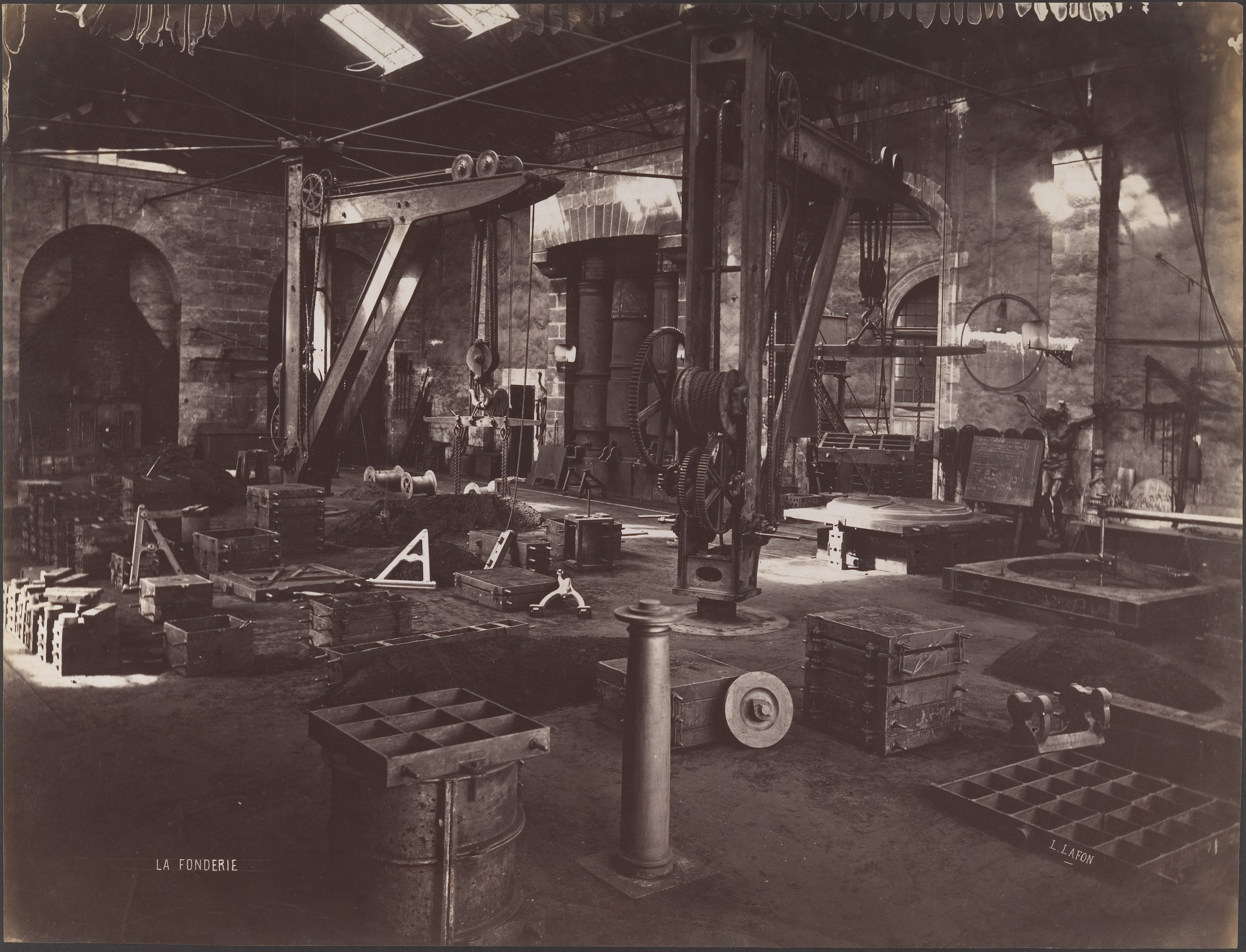This old, black-and-white photo captures the interior of what appears to be a blacksmith shop or a machine factory, characterized by its dark, murky ambiance despite some skylights. The sepia-toned image reveals an array of industrial machinery, including gears, pulleys, and cranes equipped with hooks and cables, suggesting equipment designed for lifting heavy objects. The floor, likely concrete, is strewn with wooden crates and pallets that have sections carved within them. A large metal pole protrudes from the ground in the foreground, possibly serving as a barrier or fixture. The brick walls rise to curved doorways, leading to an array of stored items, including large metal barrels stacked in the background. Centered is a steel structure with gears, potentially part of a crane system, indicating its use for heavy lifting operations. The back wall houses an unlit furnace, reinforcing the possibility of this being a blacksmith's workspace. Overlaid text on the bottom left reads "La Foundry," suggesting a foundry or metalworking establishment. The overall scene, devoid of human presence, exudes an atmosphere of antiquity and hard labor.